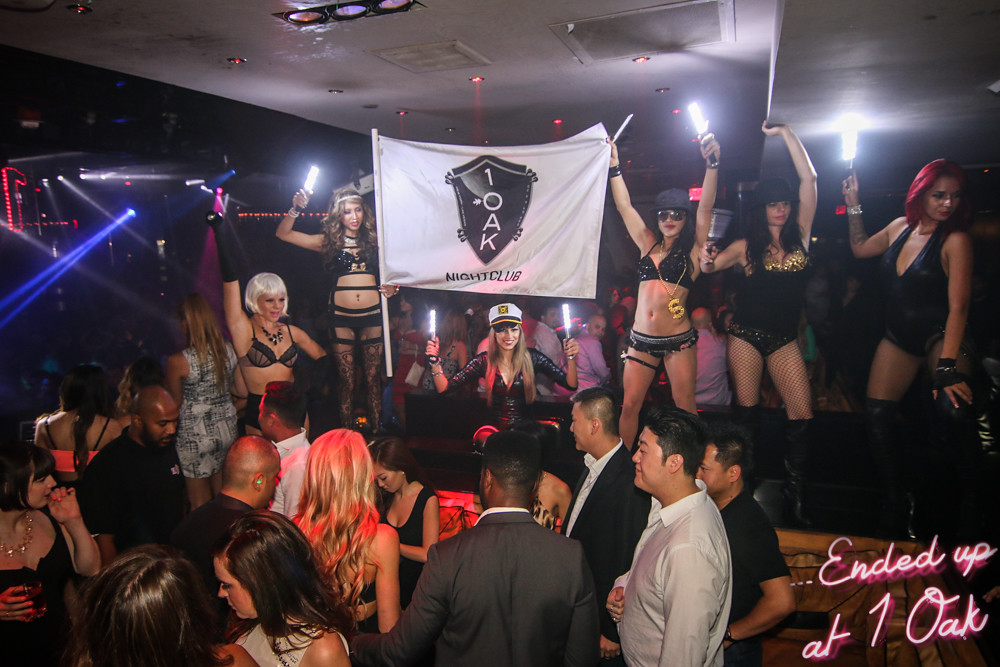This image depicts a vibrant scene inside One Oak Nightclub, illustrating a lively celebration. Centered in the photograph is a commanding figure— a woman donned in a black leather top and a captain’s hat, holding glow sticks in each hand. Surrounding her are several women, all dressed in stylish black bras, underwear, and some sporting accessories like hats, sunglasses, and stockings. Two women prominently display a white banner with a black shield emblem, emblazoned with "One Oak" in white and "Nightclub" in black beneath it. The ambience is further enhanced by a group of women, one of whom wears a large gold ‘S’ necklace, standing joyfully with drinks in hand, engaging with the crowd in front of them. In the lower right corner, the text "Ended Up at One Oak" glows in pink neon, capturing the essence of this festive night.